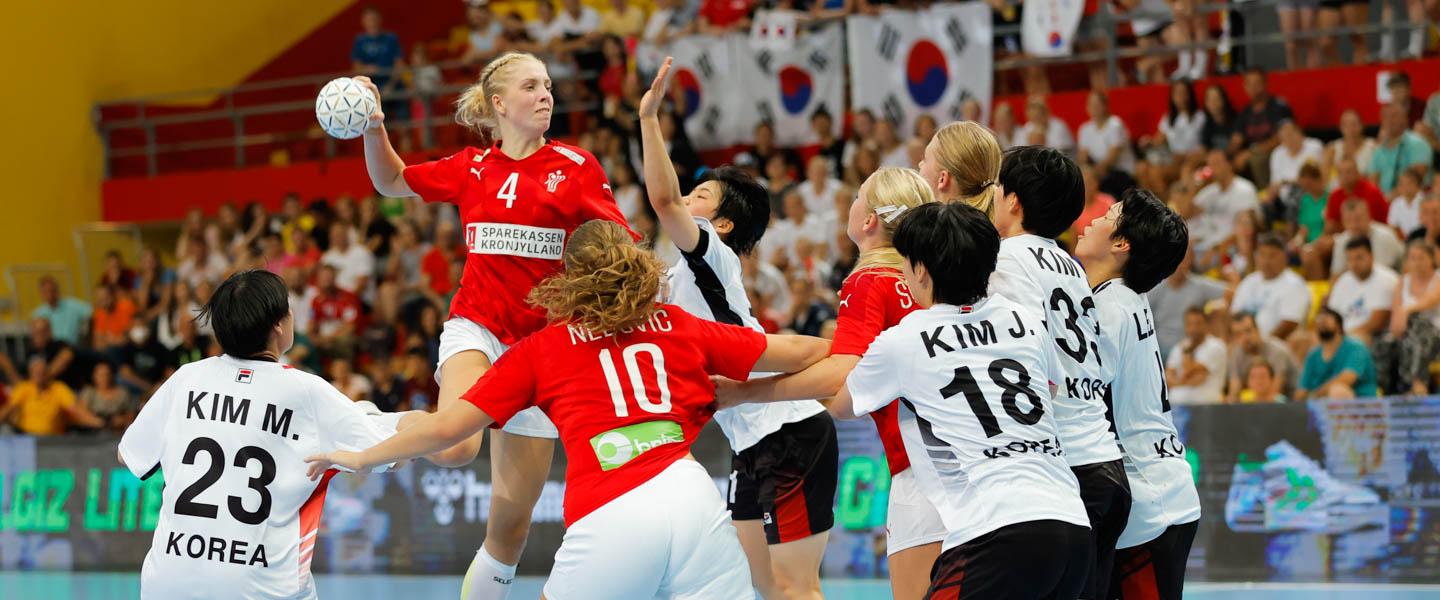The photograph captures an intense moment during a competitive game resembling handball or throw ball. Central to the action is a girl wearing a red jersey numbered 4, who is airborne and gripping a white ball with a triangular pattern, poised to make a critical play. To her right is a blond-haired girl from the same team. On the left side of the image, an opposing player from Korea, identified by her jersey reading "Kim M 23 Korea," is positioned defensively. Nearby, another player in a red jersey numbered 10 and white shorts, along with another Korean player, "Kim J 18," can be seen. The audience forms a blurred background, with several Korean flags visible atop the bleachers, underscoring the international nature of the competition. The dynamic scene is filled with motion and anticipation, reflecting the intensity of such a high-stakes game likely akin to an Olympic event.